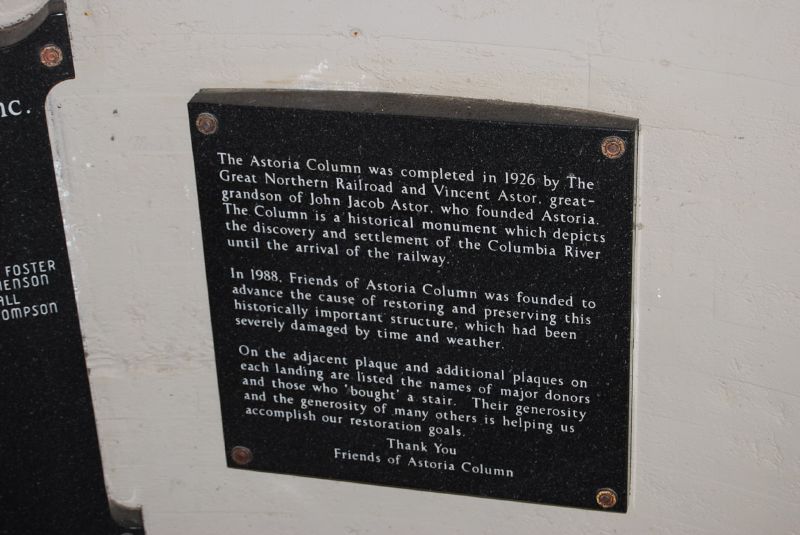The image depicts a rectangular photograph focusing on a black stone plaque with white flecks, bolted into a gray painted stone wall. The plaque is fastened at each corner with screws and features white text. It reads: "The Astoria Column was completed in 1926 by the Great Northern Railroad and Vincent Astor, great-grandson of John Jacob Astor, who founded Astoria. The column is a historical monument which depicts the discovery and settlement of the Columbia River until the arrival of the railway. In 1988, Friends of Astoria Column was founded to advance the cause of restoring and preserving this historically important structure, which had been severely damaged by time and weather. On the adjacent plaque and additional plaques on each landing are listed the names of major donors and those who 'bought a stair.' Their generosity and the generosity of many others is helping us accomplish our restoration goals. Thank you, Friends of Astoria Column." The surrounding environment is not clear, but another plaque can be seen partially visible to the left.